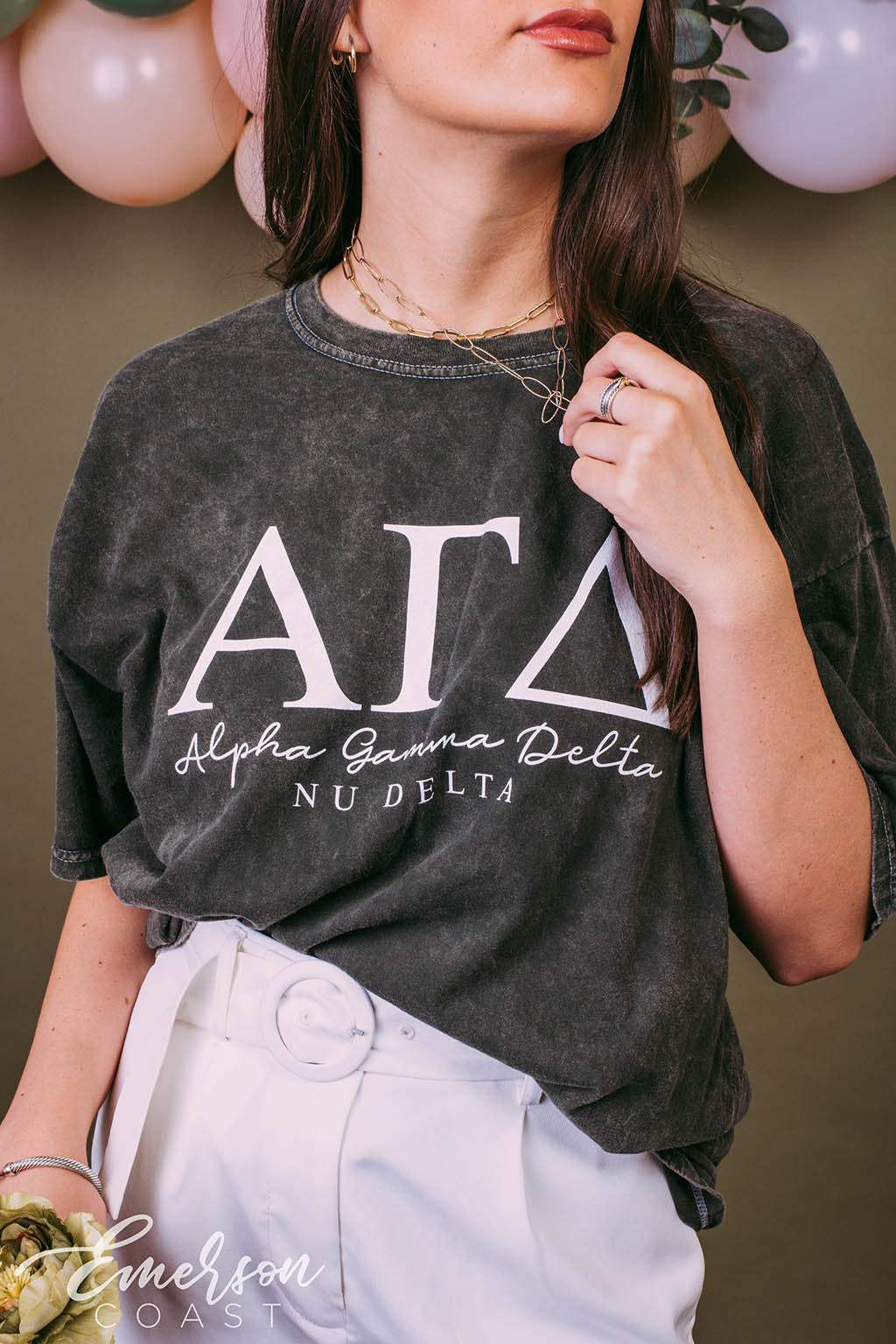In this detailed color photograph, a young woman models a dark gray t-shirt with white lettering. The image is in portrait orientation, capturing the subject from above her lips to just below her hips. She has long dark brown hair and is wearing a gold chain necklace and a silver ring on one of her fingers. Her t-shirt, emblazoned with "Alpha Gamma Delta Nu Delta" in a mix of script and block fonts, is paired with stylish white dress pants and a belt at the waist. She holds a flower in her right hand while her left hand touches her necklace. The bottom left corner of the image features the logo "Emerson Coast" in white lettering. The background is primarily gray, and behind her head are pink and white balloons. The photograph exemplifies fashion and product photography, focusing on the t-shirt associated with the sorority, Alpha Gamma Delta.